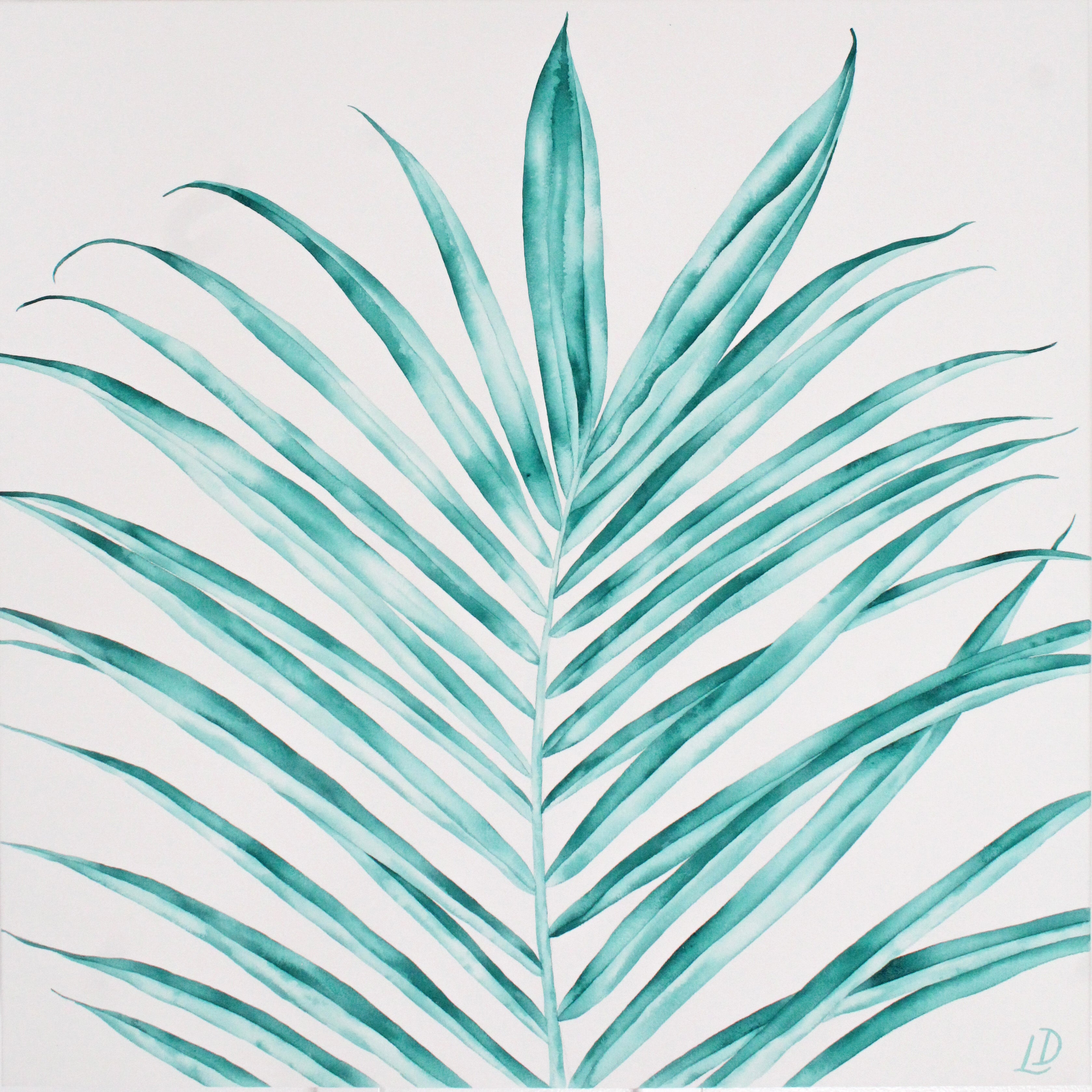The painting features a detailed depiction of a many-leafed plant rendered in watercolor style, set against an off-white, cream background. The plant's central stem, which is a light green, rises from the bottom center and arches slightly to the right, giving a sense of organic motion. From this stem, a lush array of 30 long, thick leaves emerges, with 15 on each side. The leaves display a mesmerizing blend of light green, dark green, and varied shades of teal, ranging from aqua to dark turquoise, mingled with touches of white for added depth. The top center leaves are notably the largest and most prominent. The painting almost entirely fills the square canvas, leaving only the upper corners clear. In the bottom right-hand corner, the artist's signature, "LD," is delicately inscribed in a light teal script, with the "L" slightly below the "D." The plant, with its intricate and harmonious blend of colors, suggests a type of indoor greenery, vibrant and full of life.